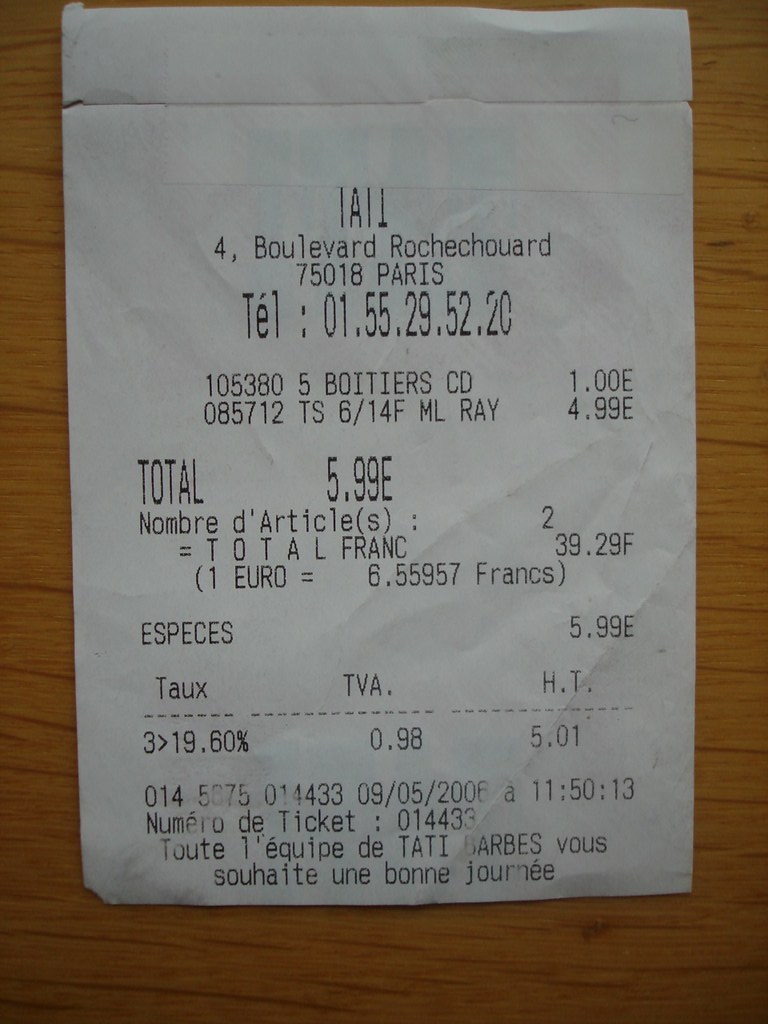The image is a detailed color photograph of a receipt placed on a wooden surface. The receipt, printed on thin white paper, is oriented in portrait mode, with the wood beneath arranged horizontally, descending slightly diagonally to the right. The wooden surface is a dark orange pine color, with dark brown grain patterns and knots adding texture and character. 

The receipt is in French, and at the top, it features the address "Boulevard Rochechouart" in the 75018 Paris area. Below the address, a telephone number is printed: "01.55.29.52.20." 

The list of purchased items includes a "Boitiers CD," priced at 1 euro, and another item described as "M.L. Ray" for 4.99 euros. The total cost for the transaction is 5.99 euros. At the bottom of the receipt, the date and time of the purchase are noted as "09.05.2006" and "11:50:13" respectively.